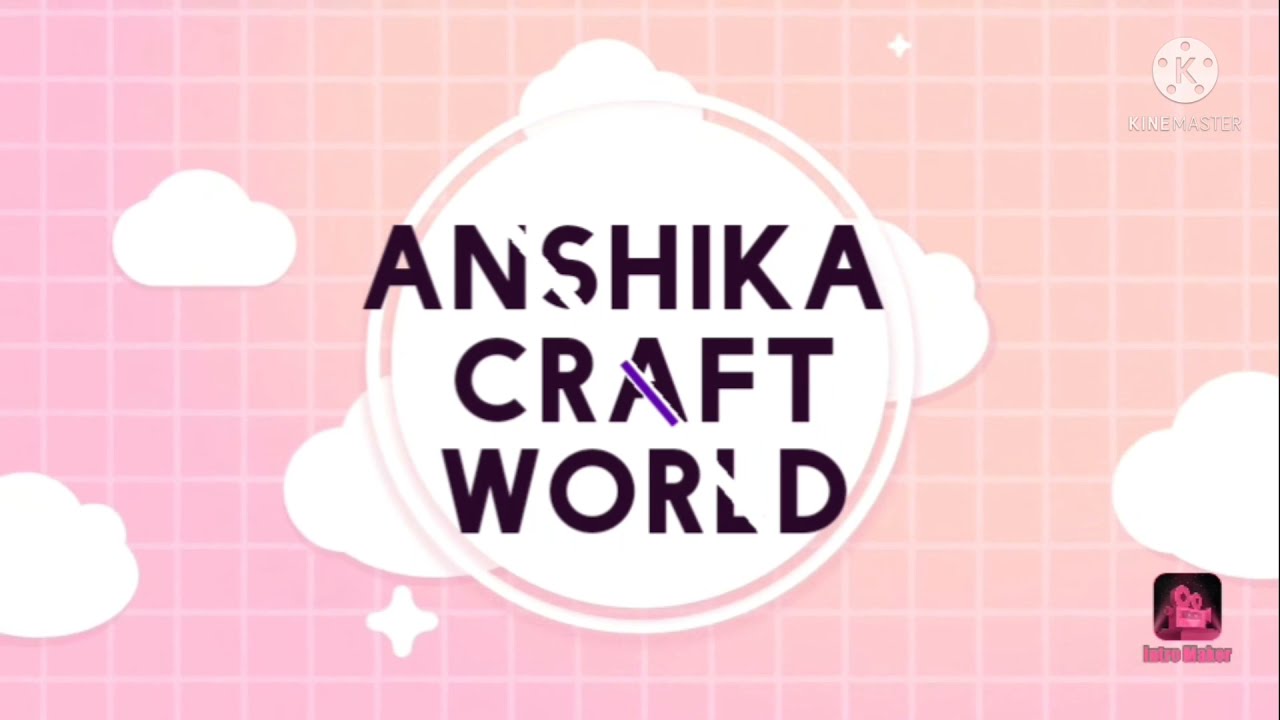The image resembles a business card with a digital design. At its center, the text "Anshika Craft World" is prominently displayed in black font on a white circular background, which has a thin white outline. The letters appear slightly erased down the middle, creating a visual streak that includes a purple line. The overall background features a gradient, transitioning from a darker, pale red on the left to a peachy hue towards the center and right. Superimposed on this gradient backdrop is a grid pattern of white lines. Additionally, there are stylized white clouds beneath the central text. In the top right corner, there's a logo with the letter 'K' inside a circle, and below it, the word "KineMaster." In the bottom right corner, there is an icon resembling an old-fashioned film projector with the word "MAKER" partially visible beneath it.